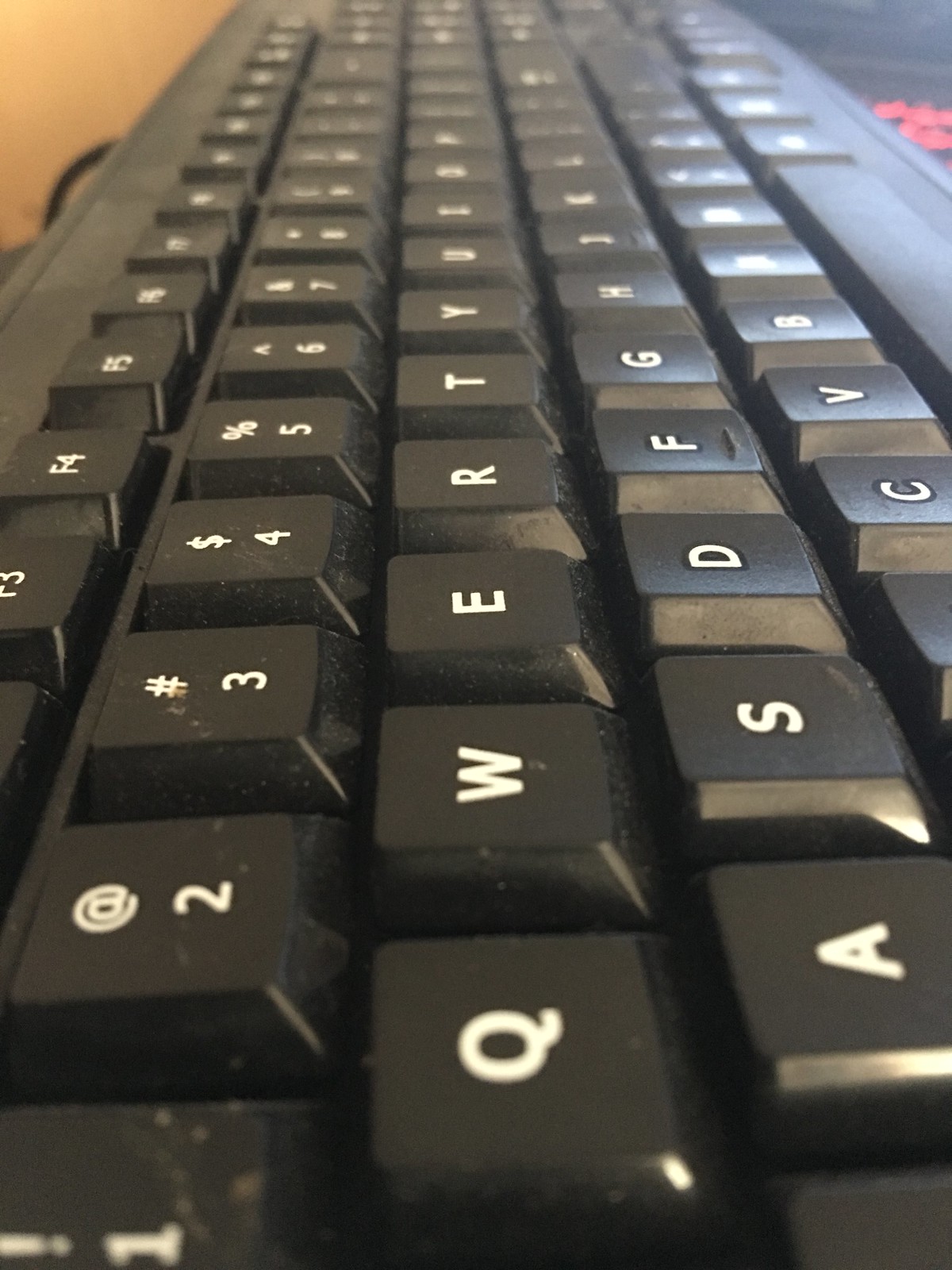The image captures an up-close, side-top view of a standard full-size black keyboard with white lettering on the keys. The photo shows at least three-quarters of the entire keyboard, with a focus on the nearest keys, revealing small bits of dust, smudging, and light brown spatters on the number keys. Despite the dirt and debris, the white lettering remains clear and unworn, suggesting the keyboard is relatively new. The background is blurred due to the close-up perspective but hints at its surroundings, showing a sandy brown or wheat-colored wall and a black cable running from the upper left side of the keyboard. Additionally, a red item is faintly visible on the top right side of the image, and the background seems to contain a light brown surface, possibly a table.